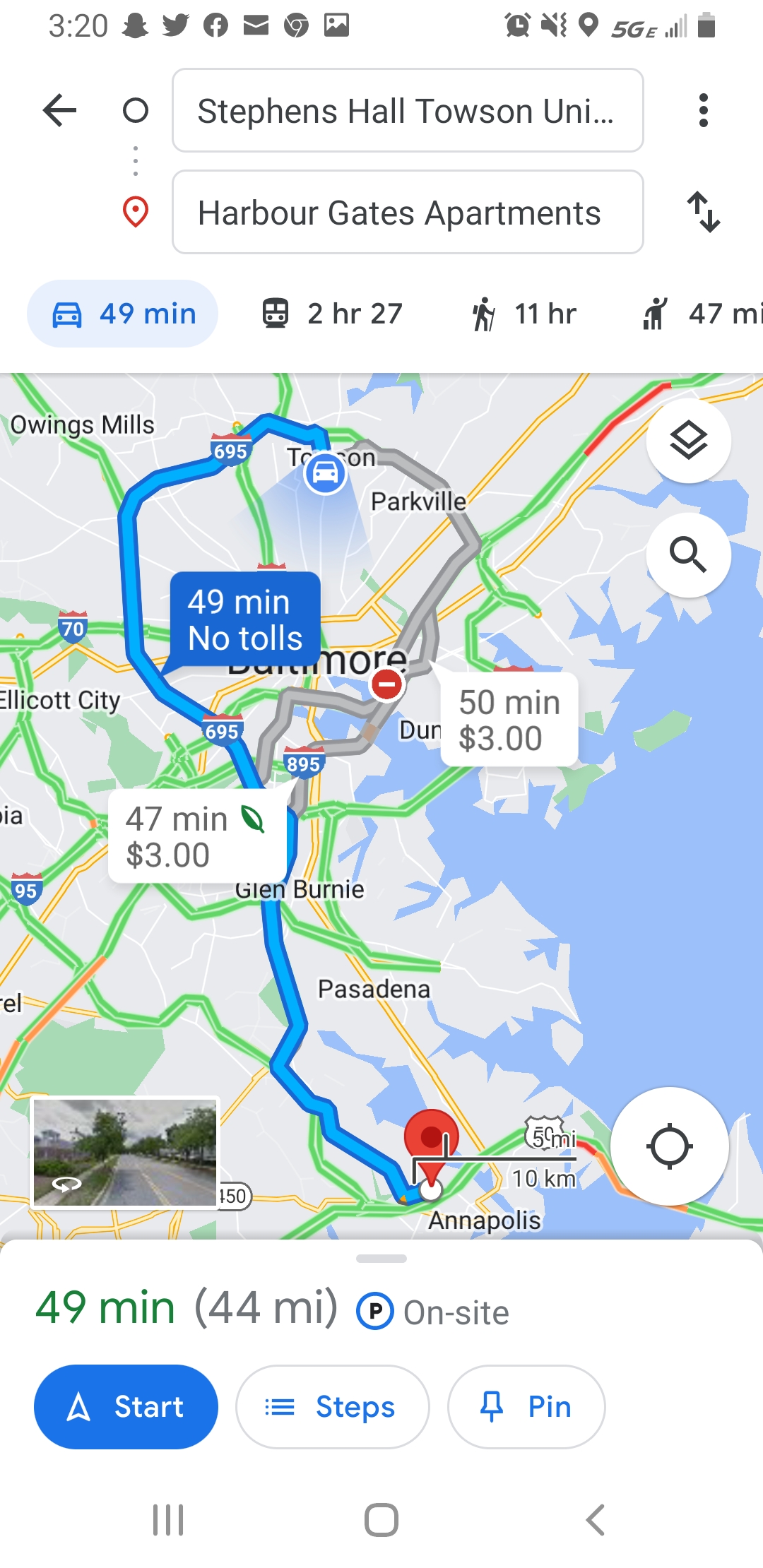The image is a screenshot from a navigation app on a smartphone. At the very top left of the screen, numerical indicators show "3", "4", and "20". Additionally, there are various app icons, including Snapchat, Facebook, email, Google Chrome, Photos, a clock, silence/vibration, a location pin, 5GE connectivity with 3 out of 5 signal bars, and a battery icon that is slightly depleted. Below this, there is a search bar indicating a destination or location, possibly "Stevens Hall, Townsend University," and another location listed as "Harvard Gates Apartments."

In the lower left of the screen, there are estimated travel times for different modes of transportation: 49 minutes by car, 2 hours and 27 minutes by bus, 11 hours by hiking, and 47 minutes by rideshare. The map displayed on the screen appears to include areas around Pasadena, Glen Burnie, Baltimore, and Parkville. To the far right, a body of blue water is visible, and at the bottom left, there's a street view thumbnail.

Central to the image is a blue navigation route starting from the top near a location marked by a car icon. The route proceeds down through 695 to Annapolis, identified by a red pin. The right side of the map suggests an alternative route taking 50 minutes, while another on the left, labeled "Econop," shows a travel time of 47 minutes. Various green roads indicate different navigation options, with travel times of 49 and 44 minutes respectively.